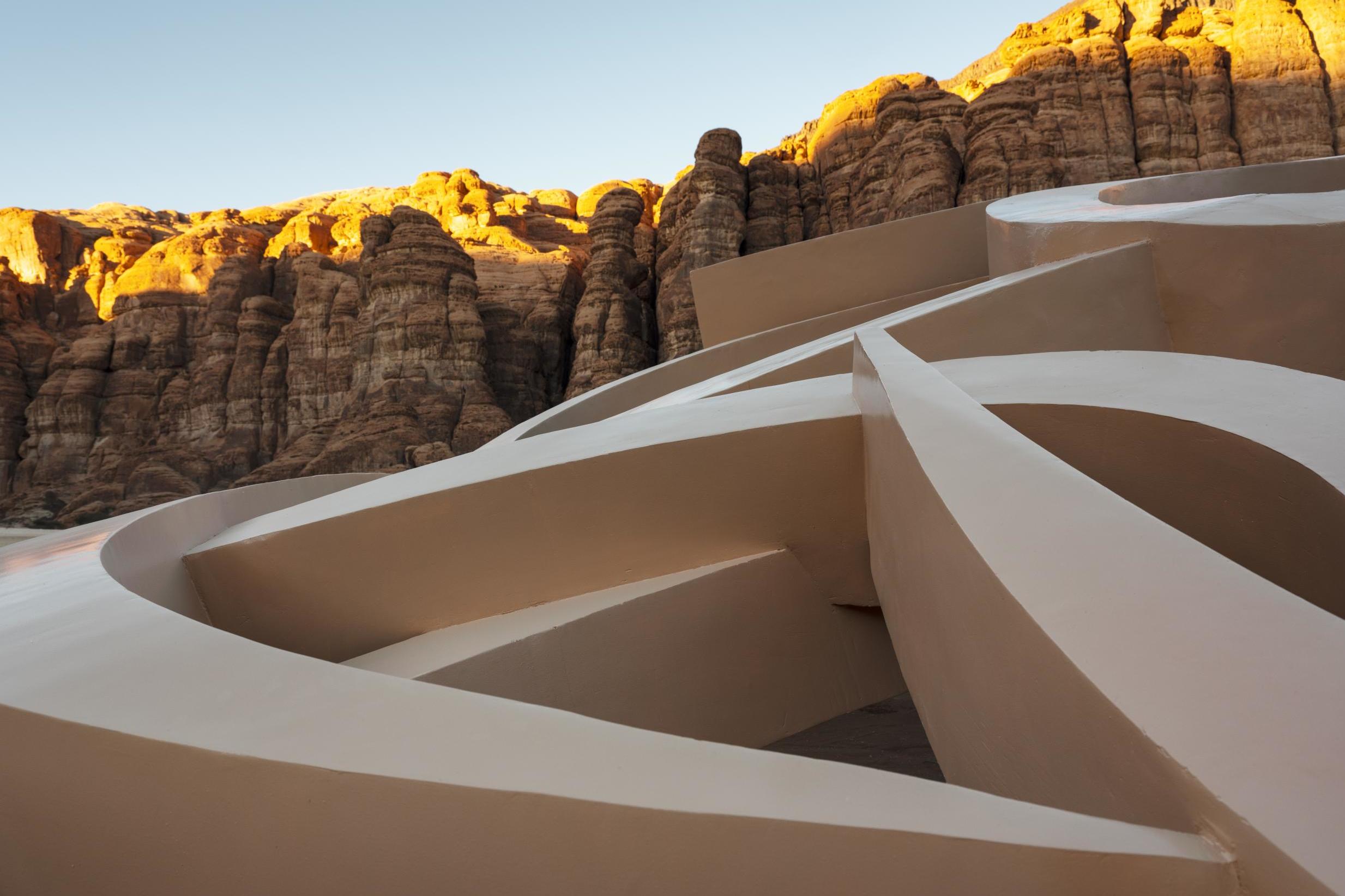The photograph captures a large, intricate sculpture known as Shifting Sands, located in an art exhibition in Jeddah, Saudi Arabia. This desert installation features a massive, three-dimensional structure made from a material resembling plaster or marble with a smooth, eggshell semi-gloss finish. The sculpture's design consists of intertwining swirls and lines that evoke the chaotic elegance of a bowl of spaghetti. The light tan color of the sculpture harmonizes beautifully with its desert surroundings. In the background, layered rocky hills, formed over countless years, add to the rugged natural beauty of the scene. The image is taken at sunrise, with the subtle morning sunlight casting a soft glow on both the sculpture and the amber-toned stone formations behind it, creating a striking contrast against the clear sky. The combination of the foreground sculpture and the textured landscape highlights the unique fusion of art and nature in this desert setting.